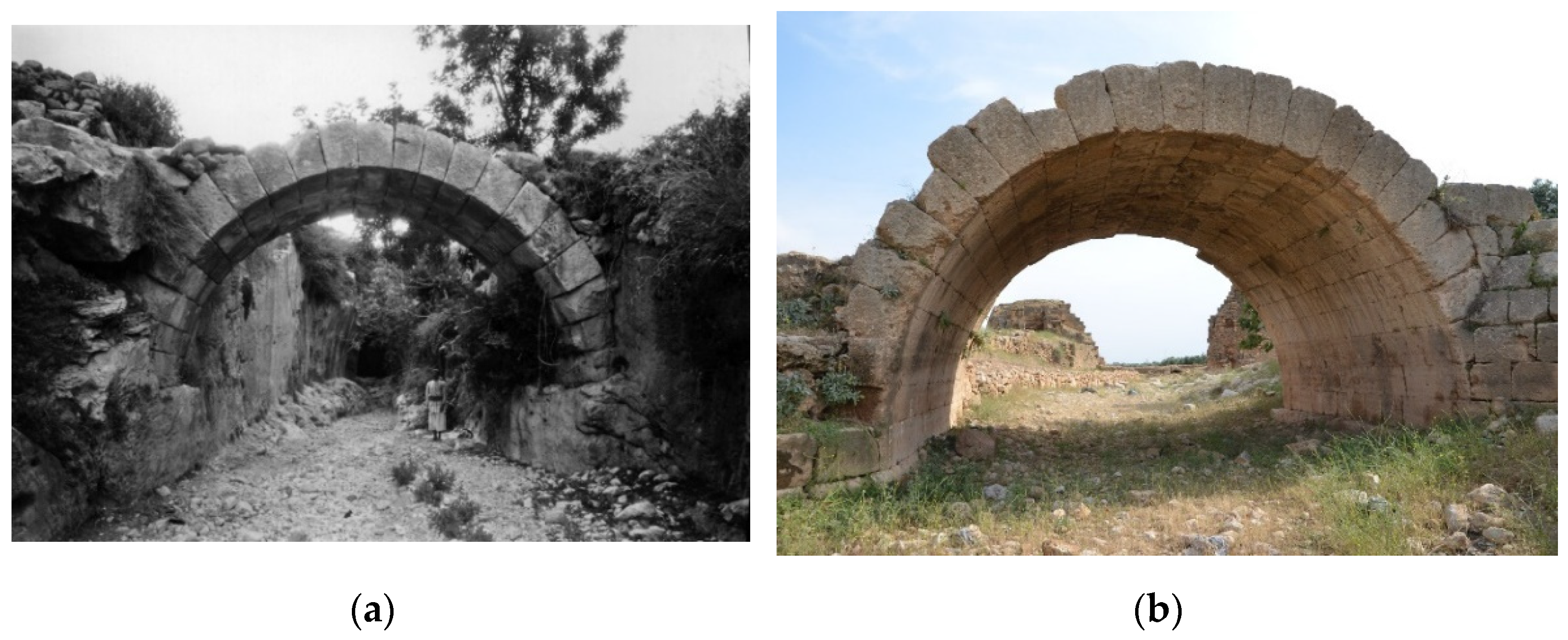This set of two photographs likely documents the same stone arch at different points in time. On the left side, labeled A in black text, is a black and white photograph of the arch. The arch is composed of stones, with a light gray stone path beneath it extending into a gravel and rocky surface. Flanking the arch are rocky surfaces, and a silhouetted tree stands prominently behind the arch against a bright gray sky. There is some visible vegetation, hinting that this area may have once been a riverbed now drained of water. 

The right photograph, labeled B in black text, presents a colored version of the arch, suggesting a more recent capture. The arch, colored light brown to gray, appears considerably weathered with overgrown grass and a stone path beneath it. The sides flanking the arch now show more gaps, with stacked stones reaching halfway up the height of the arch. Behind the arch, distant and similarly constructed stone structures are faintly visible. The landscape appears more open and devoid of the extensive vegetation seen in the left image. A white cloudy sky with a small patch of blue can be seen at the top left of the photograph.